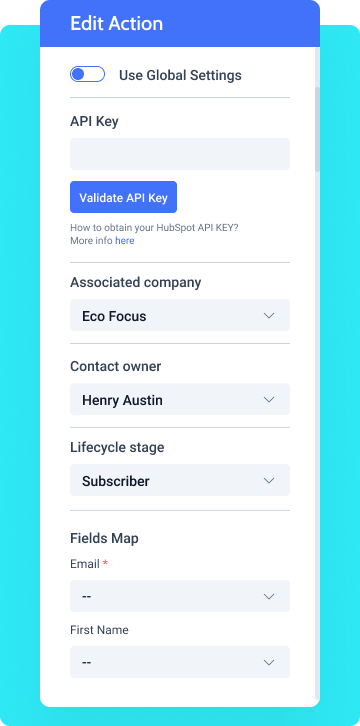This image captures a section of a website interface set against a light blue background. The top of the section prominently features the title "Edit Action." Below this title, there is an option labeled "Use Global Settings," accompanied by a blue toggle button indicating that it is currently active.

Further down, the section is broken into several informational fields. The first field is labeled "API Key," followed by a "Validate API Key" button directly beneath it. Below these elements, there is a prompt that reads, "How to obtain your HubSupport API Key?" accompanied by a question mark and a link labeled "More info here."

The next section pertains to an associated company, "EcoFocus," with further details listed: the contact owner is "Henry Austin," and the LifeCycleState subscriber is "Phil's Map." Each of these entries is paired with a drop-down menu, indicated by a small arrow to the right, allowing for additional options or information.

Finally, there is an "Email" field, marked with a red asterisk indicating a required field, beside an input box currently filled with double dashes ("--"). Following this, there is another field for "First Name," also featuring a drop-down menu for further options. The design suggests that users can interact with each field to access or modify deeper settings.

Overall, every element is structured to offer a logical flow of information with interactive components for further customization, catering primarily to users managing API settings and company-related data on the platform.